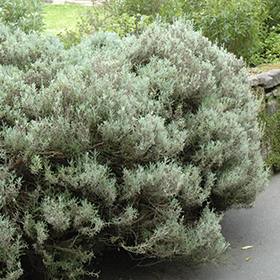In this detailed photograph, a large, bushy shrub with small, needle-like leaves is prominently featured in the foreground. The shrub, possibly quite old, is growing vigorously and extending over a pavement area that runs alongside a rustic stone wall composed of large, natural rocks. The shrub's rich green hue dominates the scene, and there are numerous branches, suggesting it might resemble a cedar bush. Beyond the stone wall, a picturesque setting unfolds with a lush green yard or park area, characterized by healthy, mature trees basking in the bright sunlight of what appears to be a summer day. In the distance, another field of green grass and a small clearing can be seen, perfectly blending with the verdant surroundings and enhancing the image's serene, nature-filled atmosphere.